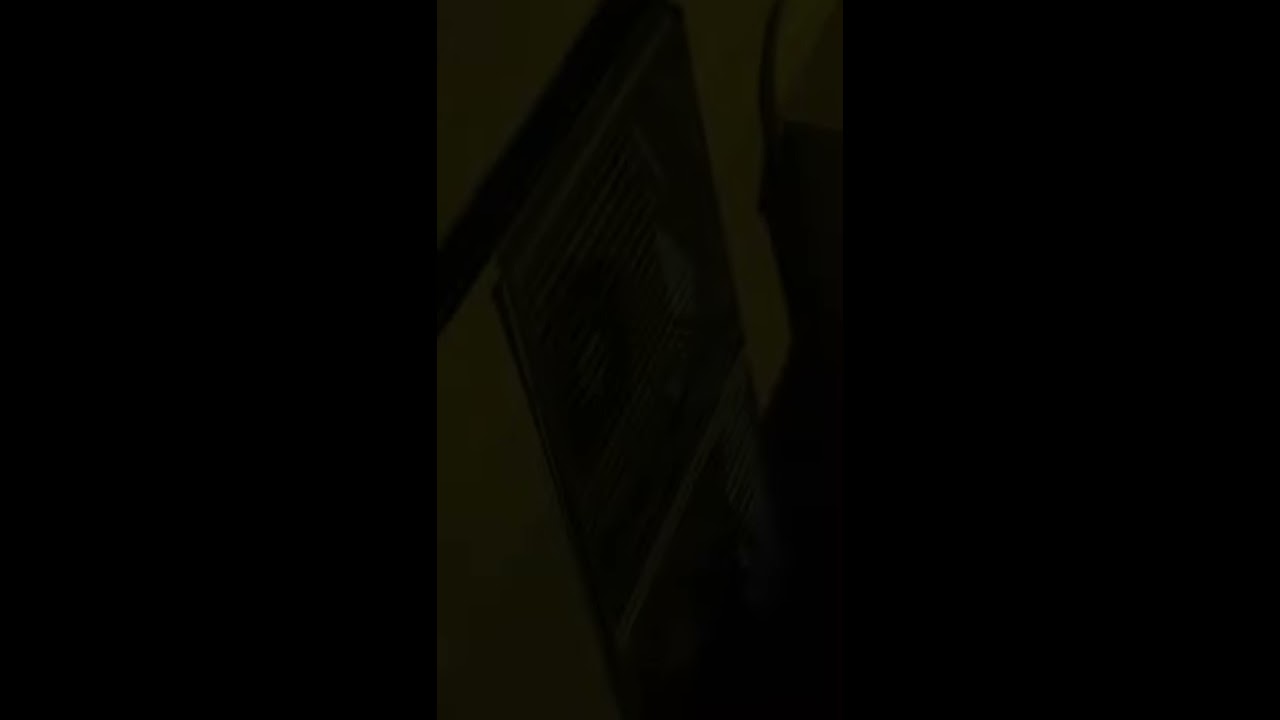This image is predominantly dark and difficult to interpret, set against a black background with thick black borders on the left and right sides. At its center, there's an olive green rectangle featuring abstract artwork that includes various shapes and lines. A black diamond shape is prominent in the middle of this green rectangle, intersected by a thick horizontal line stretching from the bottom left to the upper middle section. Additionally, within the green section, there's another diamond shape partially cut off at the bottom right, and a curved shape on the right side resembling a full-length apron. The overall impression is one of murky, intricate graphics that are hard to define precisely due to the image's dark and obscure nature.